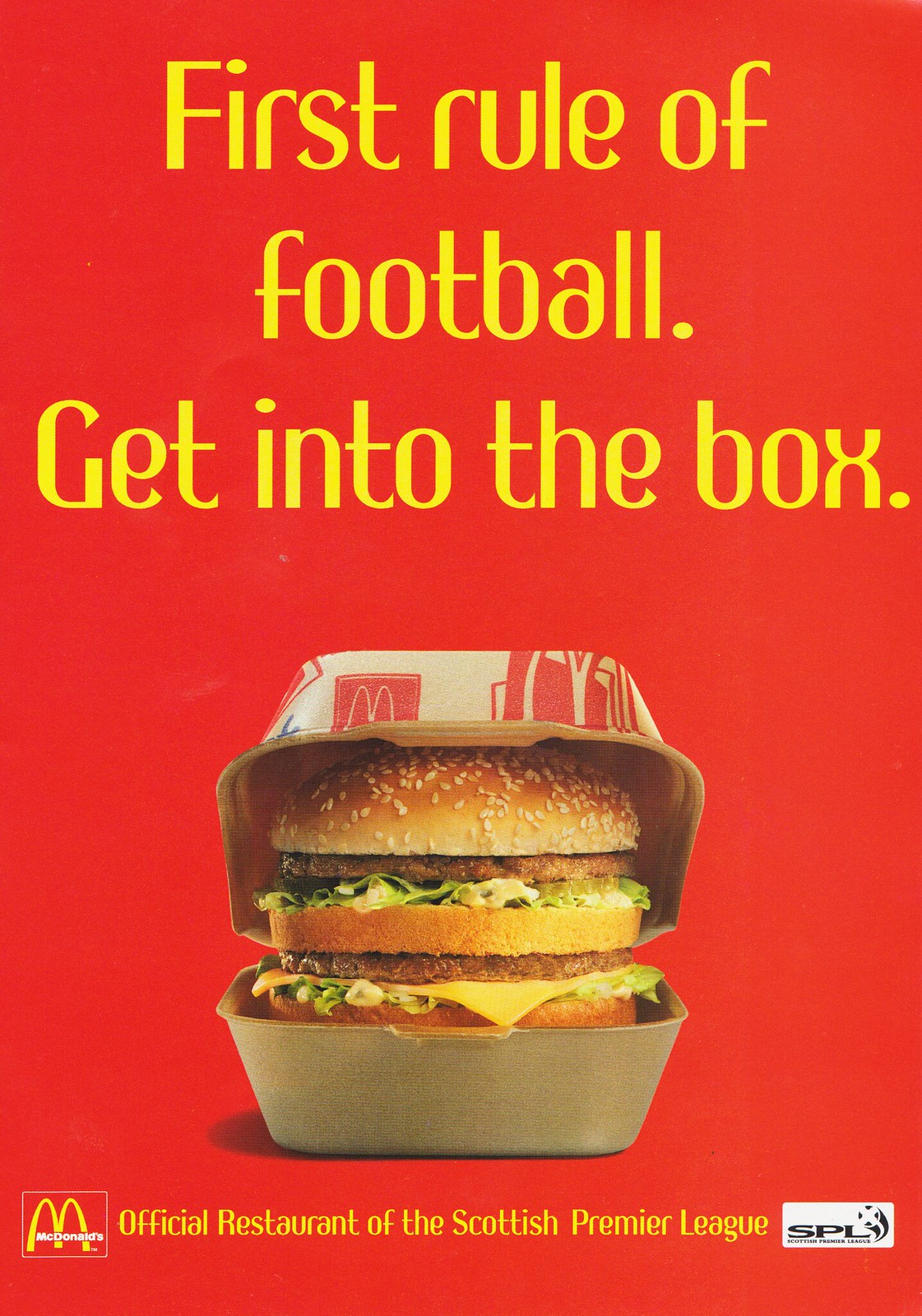This advertisement for McDonald's and the Scottish Premier League features a striking red background, typical of McDonald's branding colors. Prominently displayed in the center is a Big Mac inside an open, light-brown cardboard box. The Big Mac boasts a sesame seed bun on top, three layers of bread, two beef patties, cheese at the bottom, and layers of lettuce in between. The McDonald's arch logo appears repeatedly on the box lid, underscored by a red square with a stylized brown "M".

At the top of the ad, in bold yellow text, the slogan reads, "First rule of football, get into the box," making a playful connection between soccer terminology and the burger packaging. Below the box, the familiar McDonald’s logo appears on the bottom left—a red square with a yellow "M" and "McDonald's" in white text. The bottom center of the ad states, "Official Restaurant of the Scottish Premier League," linking the fast-food giant with the popular football league. To the right of this text is the SPL logo in a white rectangle, accompanied by a black-and-white soccer ball with motion lines, emphasizing the ad’s sports theme.